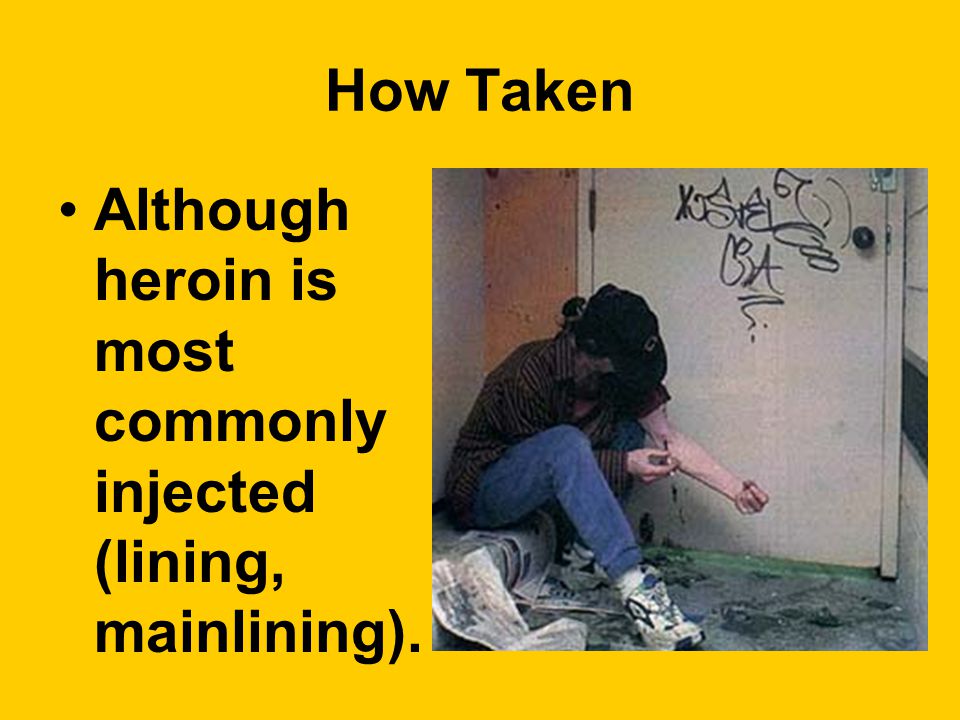The image features a striking composition with a bright yellow background. Centered within the frame is a poignant photograph of a person injecting heroin into their arm. The individual, sitting on a concrete step beside a graffiti-covered door, is immersed in a scene of urban decay marked by scattered crumpled newspapers. The person, whose gender appears ambiguous due to conflicting descriptions, wears a black shirt, blue jeans, and white sneakers, along with a dark hat—possibly a Chicago Bears hat. The individual's posture, with a needle poised at their arm and their face turned downward, conveys the gravity of the moment.

Text overlays the image, enhancing its narrative. At the top, in bold black letters, it reads "How Taken." On the left side of the photograph, additional black text provides informational context: "Although heroin is most commonly injected," with the terms "lining" and "mainlining" noted in parentheses. This detailed depiction serves as both an explicit portrayal of heroin use and an educational piece about substance abuse.